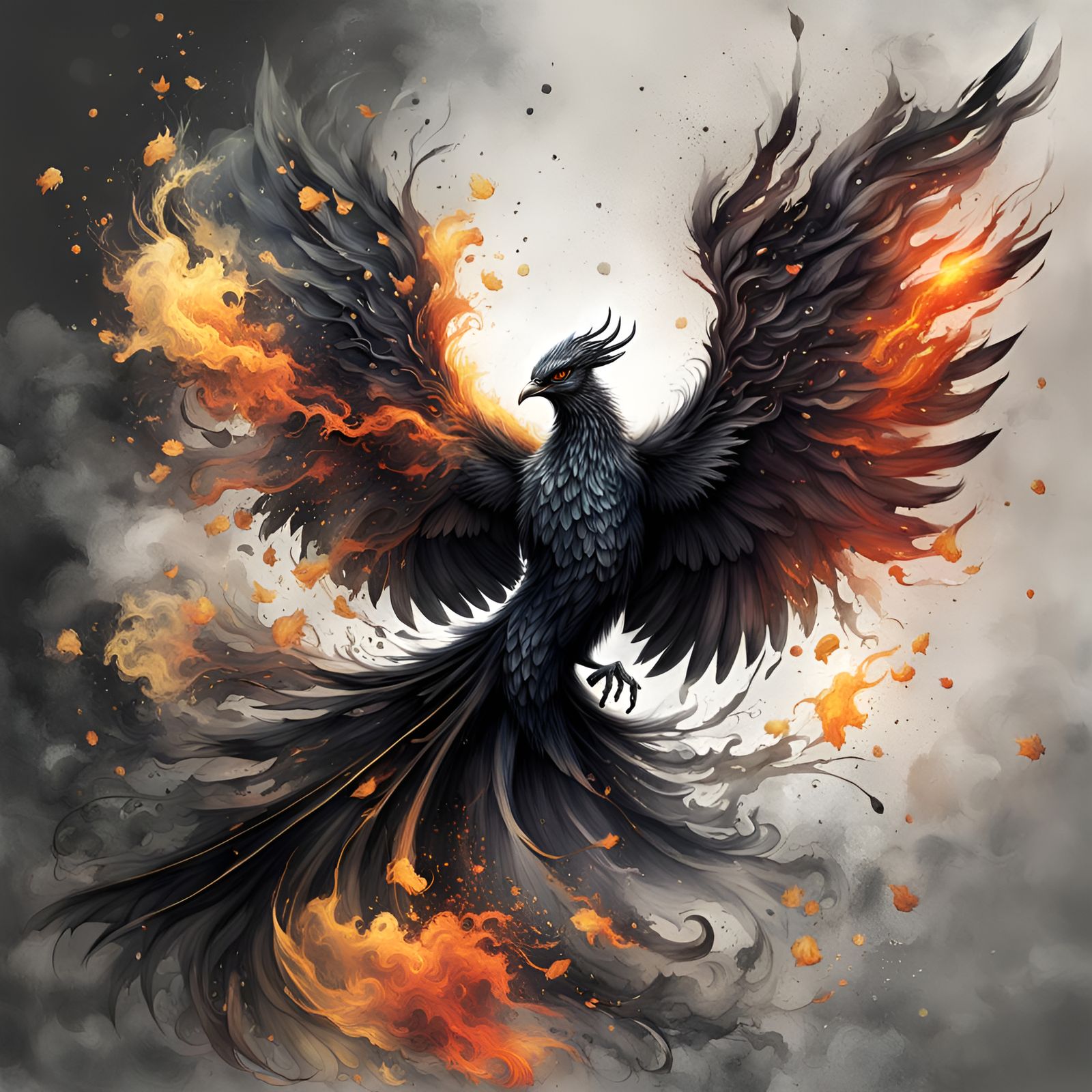This square, borderless artwork portrays a striking, multi-colored phoenix set against a background of swirling grey, white, and black smoke. The bird itself is primarily black with dark charcoal and brownish-colored feathers, and it has vivid red eyes and a yellow beak. Its feather crown adds to its regality. The phoenix's wings and extensive tail feathers are spread wide, giving the impression of powerful flight. Flames emanate from its wings and tail feathers, with orange tongues of fire shooting off into the smoky air. The background of dark and light grey clouds frames the bird, enhancing the dramatic, almost stormy atmosphere. The entire scene conveys a sense of alertness and enormity, with no text or artist signature visible.